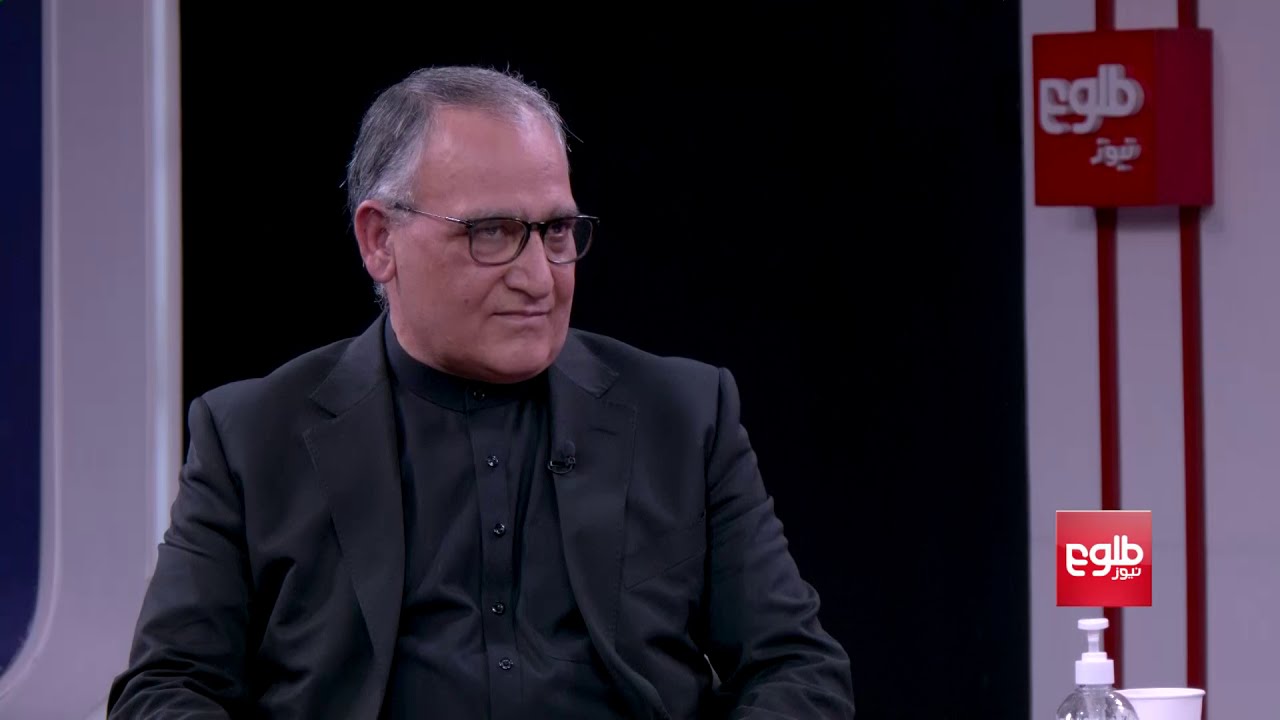The image depicts an older gentleman prominently positioned in what appears to be a studio interview or a conference setting. He is wearing a black button-up shirt paired with a black blazer. His thinning gray hair complements his receding hairline, and he is sporting thin-framed glasses with silver arms. A microphone is pinned to his lapel, and his expression appears irritated or stern as he looks off to his left. The backdrop is predominantly black, with a large black rectangular section directly behind him, flanked by distinct features on both sides. On the right, there is a gray wall with two vertical red stripes; at the top of this wall, a red box displays the letters "EGLB" along with some additional white text. A desk or table in front of him holds a few items, including a hand pump bottle, likely hand sanitizer, and a white cup. The left of the backdrop has another darker section with some white and blue details. The overall setting conveys a formal tone, potentially a serious discussion or presentation.